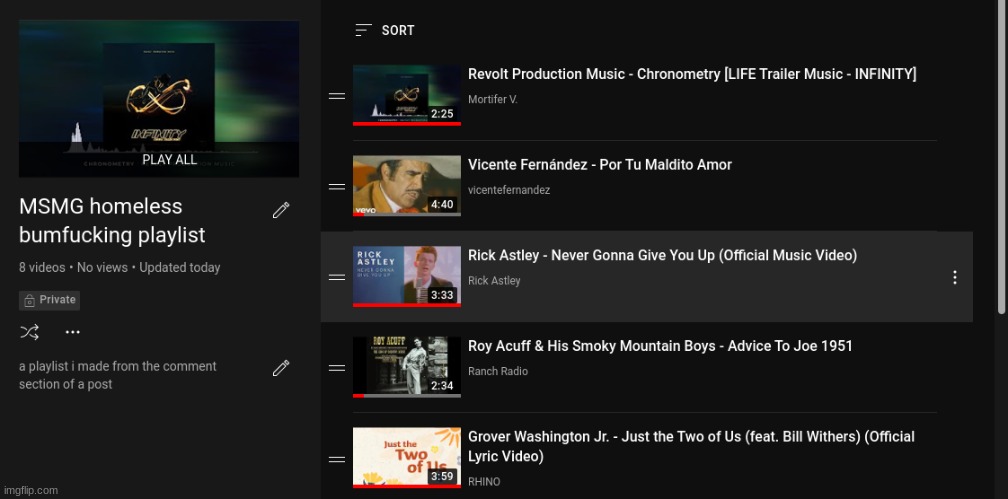This image showcases a YouTube playlist with a black background. In the upper left corner, there is a "Play All" button. Below this button, the title "MSMG Homeless Bum F***ing Playlist" is displayed in the largest text on the page. 

To the right of the title, there is an icon of a pencil. Directly below this, it states "8 videos, no views, updated today." Adjacent to this section is a box with a padlock icon, indicating that the playlist is private. Below the padlock, there's a description that reads, "A playlist I made from the comment section of a post," accompanied by another pencil icon.

In the bottom left corner, it says "imgflip.com." On the left side of the page, there is an option to sort the playlist. Beneath this, there are screenshot thumbnails for five different videos or songs that are part of the playlist:

1. The first thumbnail features a dark image with a gold-colored design, captioned with "2:25." It lists "Revolt Production Music, Chronometry, Lifetrailer Music Infinity, Mortifer V."
2. The second thumbnail showcases an image of a man with a mustache and is labeled "Vicente Fernandez, Por Tu Maldito Amor." Beneath it, it says "Vicente Fernandez."
3. The third thumbnail displays an image with the text "Rick Astley" on the side and features a man singing. It reads "Rick Astley, Never Gonna Give You Up, Official Music Video, Rick Astley."
4. The fourth thumbnail shows a man and is captioned "Roy Yakov and his Smoky Mountain Boys, Advice to Joe 1951, Ranch Radio."
5. The fifth and final thumbnail shows an image with the text "Just the Two of Us" in front of a sun. It reads "Grover Washington Jr., Just the Two of Us Featuring Bill Withers, Official Lyric Video, Rhino."